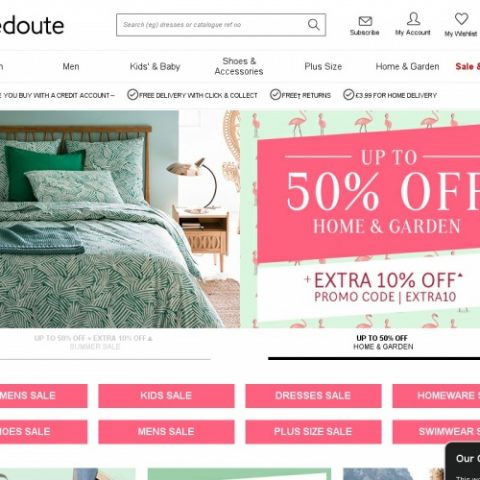This is a detailed description of a screenshot from a shop's homepage. 

At the top of the page, there is a partial title displayed against a white background, with only the letters "D-O-U-T-E" visible, suggesting the full title is cut off on the left. To the right of the title, there is a search bar with a gray outline, containing placeholder text such as "search, e.g. dresses or catalog". Next to the search bar, there are several illegible words. Further to the right, there are three icons: a letter icon labeled "Subscribe," a person icon labeled "My Account," and a heart icon labeled "My Wish List."

Below these elements, a navigation menu lists several categories: "Men," "Kids and Baby," "Shoes and Accessories," "Plus Size," "Home and Garden," and "Sale," with the word "Sale" highlighted in red. 

Under the navigation menu, a few lines of promotional text are present, though partially cut off on the left. The visible text includes: "You buy with a credit account," followed by a checkmark icon, "Free delivery with Click and Collect," another checkmark, "Free returns," another checkmark, and "€3.99 for home delivery."

Below this text, there are two images. On the left, there is a photograph of a bed, predominantly featuring green tones and leafy print patterns on the comforter. To the right, there is a graphic design with pink flamingos on a mint green background, overlaid with a pink banner that states "Up to 50% off Home and Garden." Below this graphic, in a white box with red text, it states "Plus extra 10% off with promo code EXTRA10."